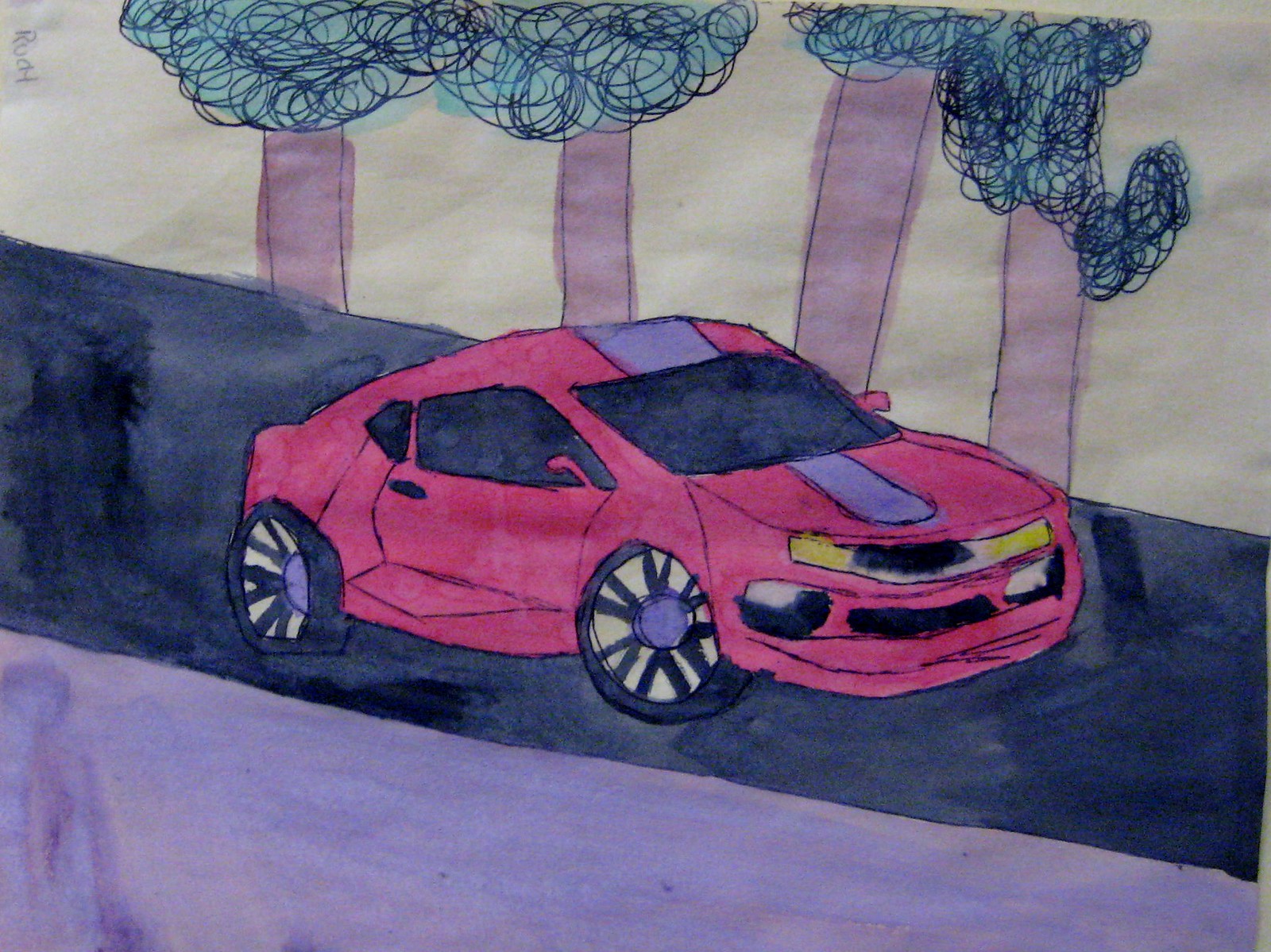This child-like hand-drawn colour illustration depicts a red sports car, prominently placed in the centre. The car is depicted from a diagonal front angle, showing the left profile across the bonnet and part of the roof. Outlined initially with pen and pencil, it is filled in using watercolour paints, evident from the soaked-in areas and dried watermarks. The car features a grey stripe from the front of the bonnet, extending over the roof ridge, and fully blacked-out windows. The wheels sport black spokes with yellow in between, set against black rubber tyres. Notably, the right rear tire appears flat.

The car is positioned on a black and grey striped road. In the background, four crudely drawn trees rise with unsystematically painted brown trunks and bushy tops created with heavy black pen swirls and filled in with green. Additional blue elements wash over parts of the image, aligning with what appears to be a blue road and other blue highlights. Atop the left side of the image, the word "road" is written vertically, emphasizing the setting. The simplistic and whimsical style, suggestive of a child’s handiwork, brings a charmingly naive view to the drawing.